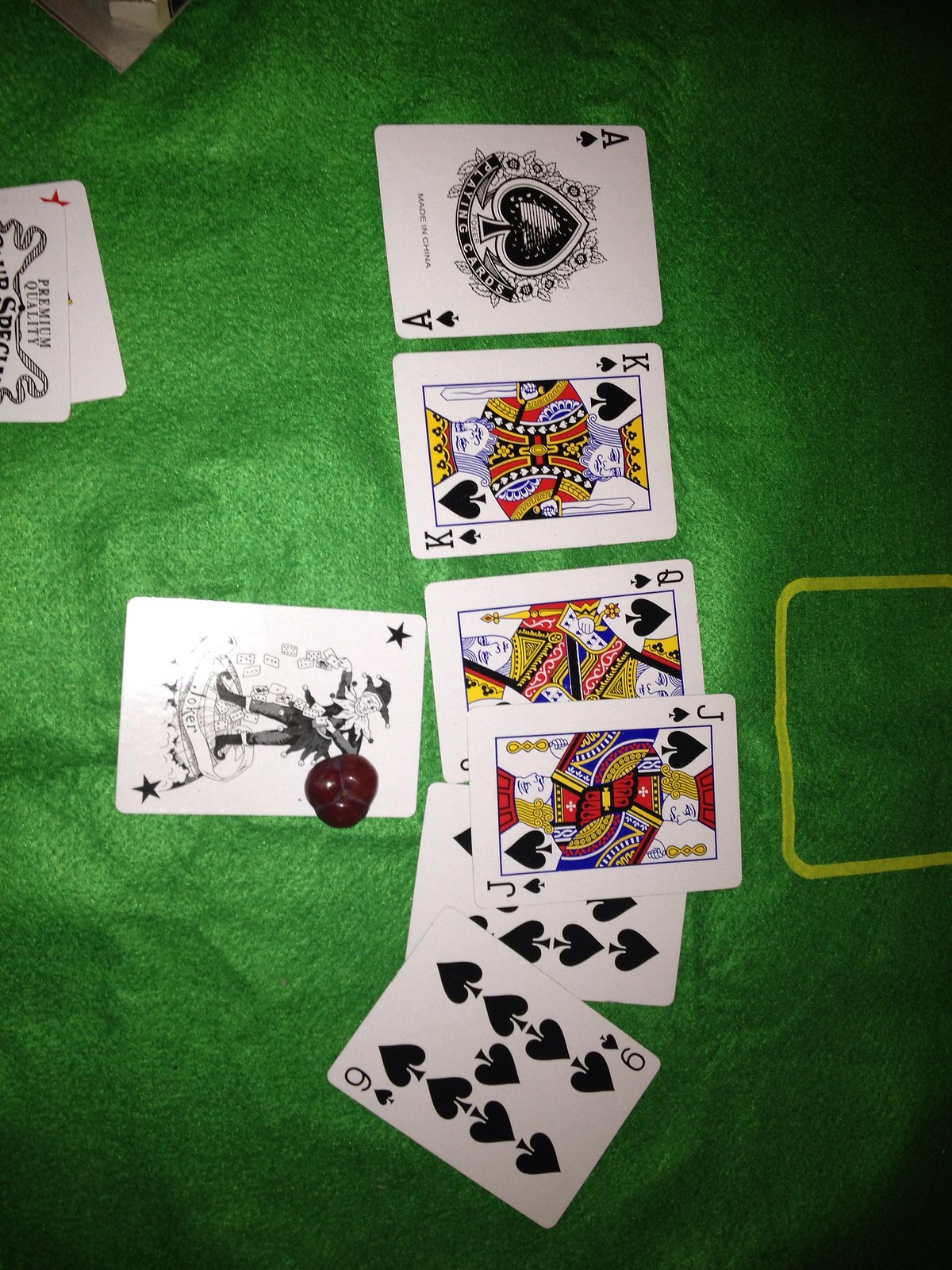The image showcases a fan of playing cards held vertically with their faces oriented towards the left. From top to bottom, the sequence begins with the black ace of spades, followed by the black king of spades, the black queen of spades, and the black jack of spades, which slightly overlaps the queen. Beneath the jack, a card with an obscured number is likely the ten of spades. The next visible card is the nine of spades. In front of the queen of spades is a black and white joker card decorated with stars in two corners, topped by an indistinct brown piece, possibly a gaming token. To the far left of the joker card, near the edge of the image, two additional cards are partially visible, though their suits and values remain hidden. The cards rest on a crinkled green surface, with part of a yellow rectangle imprinted on the fabric visible along the right edge of the image.